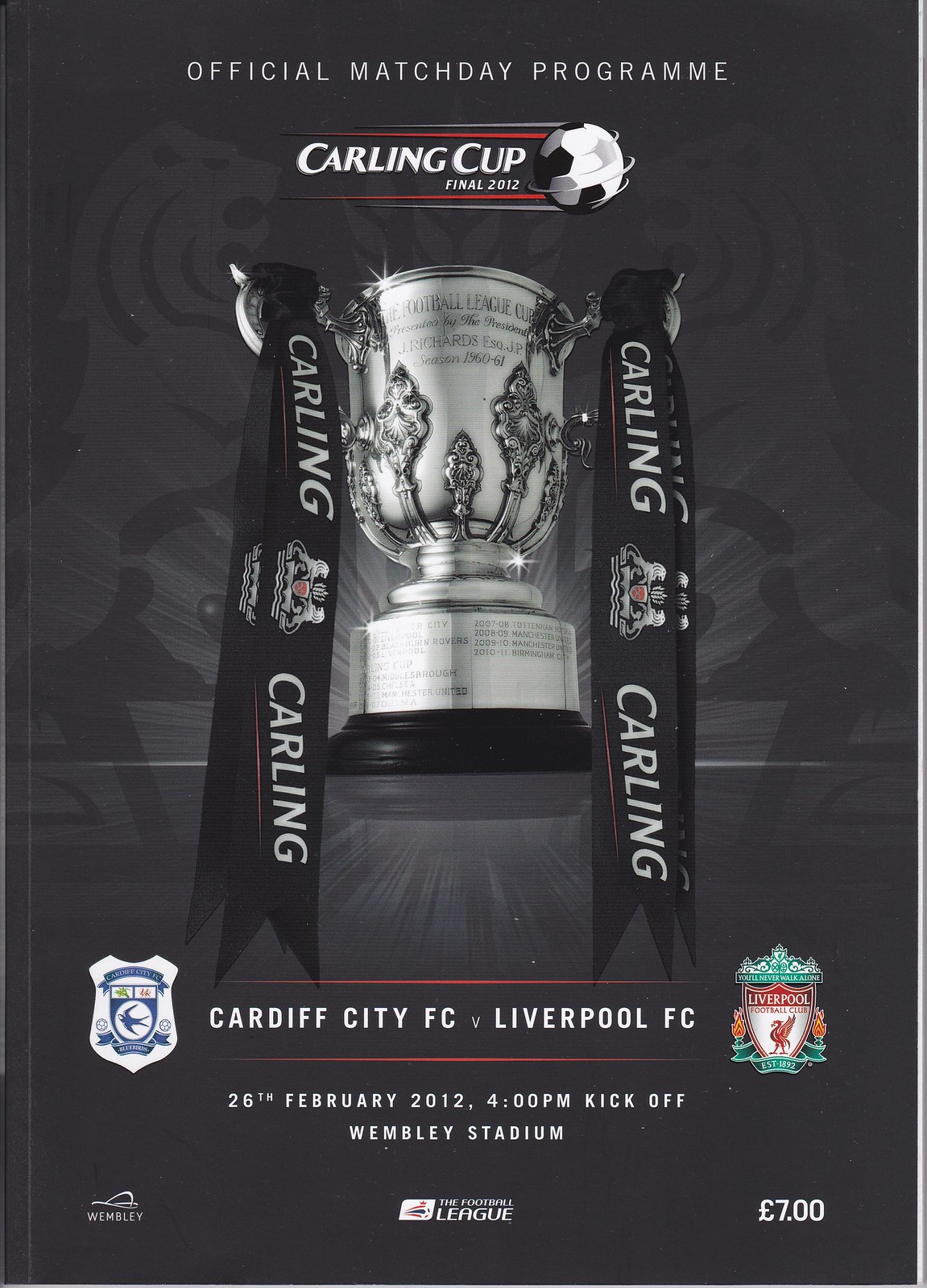The image depicts the official match day program for the Carling Cup Final 2012, featuring a strikingly detailed, shining silver trophy adorned with black ribbons that read "Carling." The background is predominantly black with subtle, indistinct designs that may resemble a tiger or lion. At the top of the poster, "Official Match Day Programme" is prominently displayed, beneath which "Carling Cup" and a dynamically swirling soccer ball can be seen. Below the cup, the details of the match are clearly outlined in white text: "Cardiff City FC vs Liverpool FC, 26th February 2012, 4:00 PM Kickoff, Wembley Stadium." Additional logos for Wembley and the Football League are positioned at the bottom, along with the price of the program listed as 7 euros.